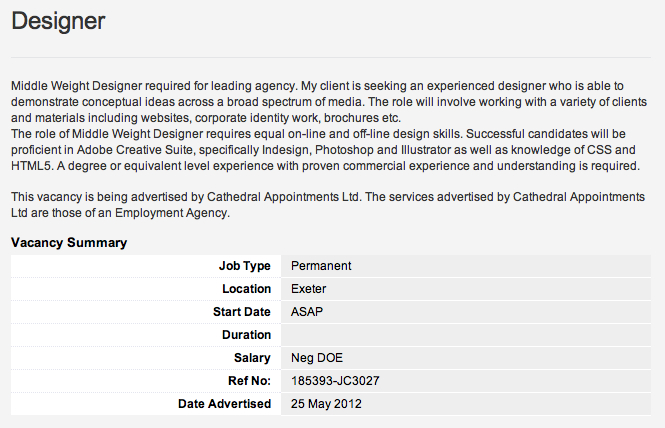The image features a light gray rectangle with black print, prominently displaying a detailed job advertisement. In the upper left corner, the word "Designer" is printed in large, bold letters with a capital 'D'. Below this, there's a thin gray line separating the header from the body text. The main text starts with the phrase "Middleweight Designer required for leading agency," explaining that the agency seeks an experienced designer adept at demonstrating conceptual ideas across various media. 

The role entails working with diverse clients and materials, including websites, corporate identity projects, brochures, and more. The successful candidate must have equal proficiency in both online and offline design skills, with a strong command of Adobe Creative Suite, particularly InDesign, Photoshop, and Illustrator.

Further down, another segment of the text includes a bold-headed section reading "Vacancy Summary." Beneath this title, there are two columns comprising seven rows each. The left column features bold black text on a white background, while the right column has regular black text on a gray background, providing a clear and organized summary of job details.